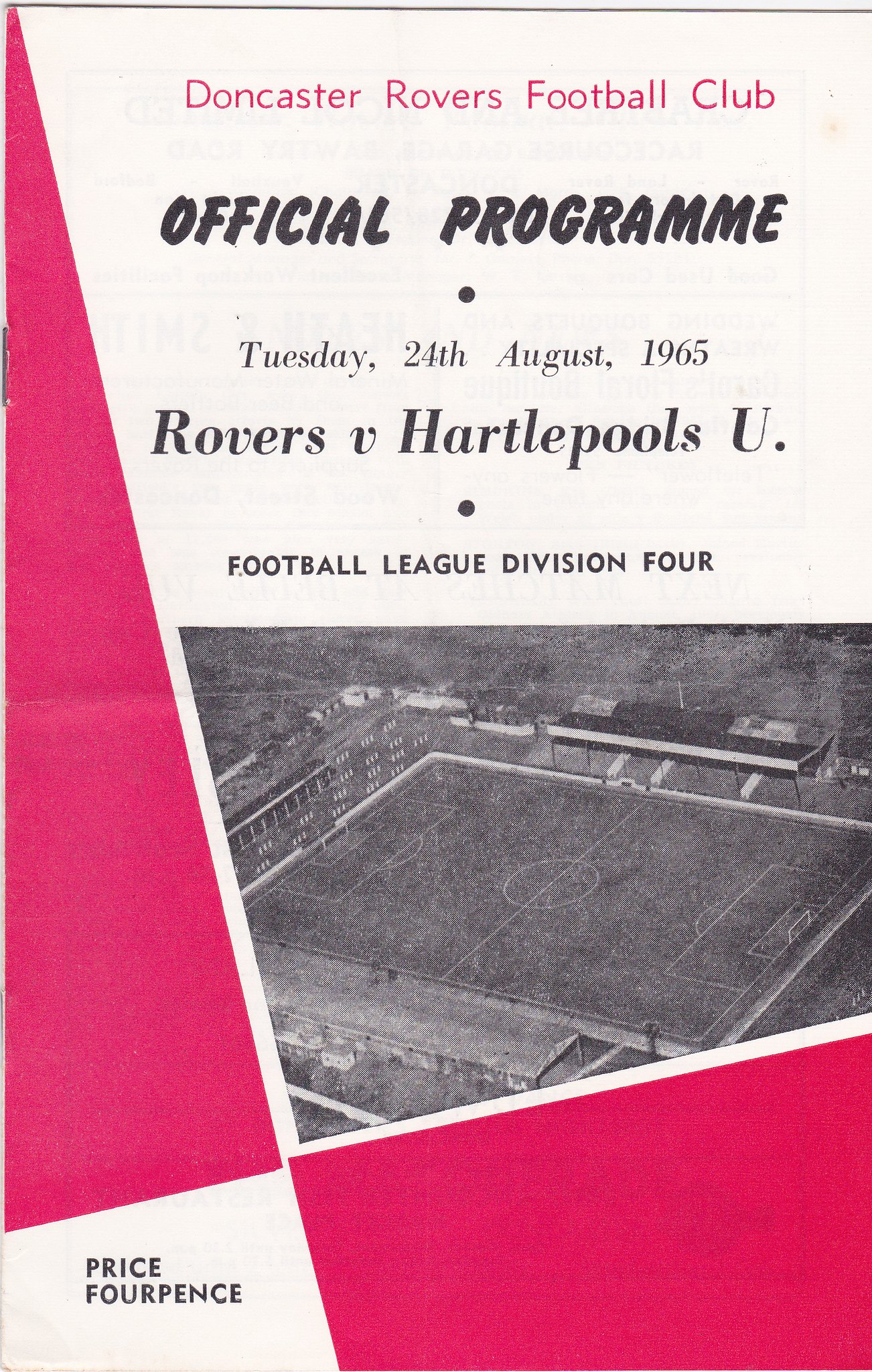This is a vintage program cover for a football match, featuring a design with a multicolored background dominated by white and bright pink elements. At the top, "Doncaster Rovers Football Club" is prominently displayed in bright pink text, followed by a bold black heading that reads "Official Program." Below this, the details of the event are provided: "Tuesday, 24th August, 1965," with "Rovers vs Hartle Pools U" and "Football League, Division IV." The price of the program, marked as "four pence," is noted in the bottom left corner. The design includes a long pink triangle from the top left, ending just above the bottom border, and a trapezium-shaped pink area in the bottom right corner. In the center, a black and white, very faded photograph of a sports field is displayed, depicting a distant view of the football ground and its surroundings.